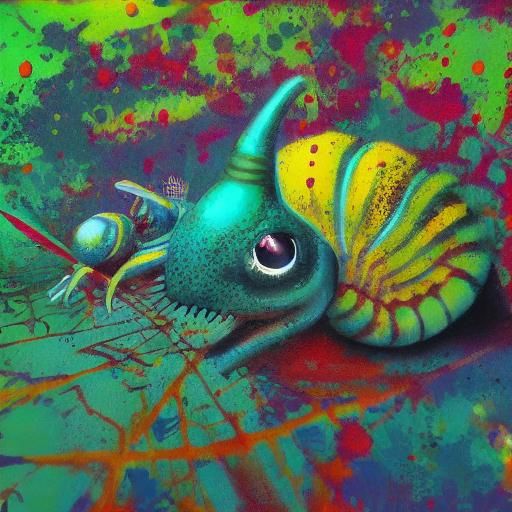The image is a vividly detailed, psychedelic artwork featuring an otherworldly insect-like creature that resembles a snail. The central creature has a neon, greenish-blue body with bright yellow and red striped segments, topped with a large, expressive black-and-white eye that gazes directly at the viewer. Its menacing face showcases sharp teeth and a striking blue horn protruding from the top of its head. This creature carries a segmented yellow shell accentuated with blue lines, further enhancing its vibrant appearance. The background is a cacophony of neon colors, including splatters and splotches of blue, aqua, bright green, red, and orange, creating a chaotic and surrealist atmosphere. Another less-defined creature or insect seen behind the main figure adds to the surreal and abstract nature of the piece. The image is reminiscent of a nuclear fallout landscape, with the intense lime green and blood-red hues contributing to its fantastical and slightly eerie ambiance.